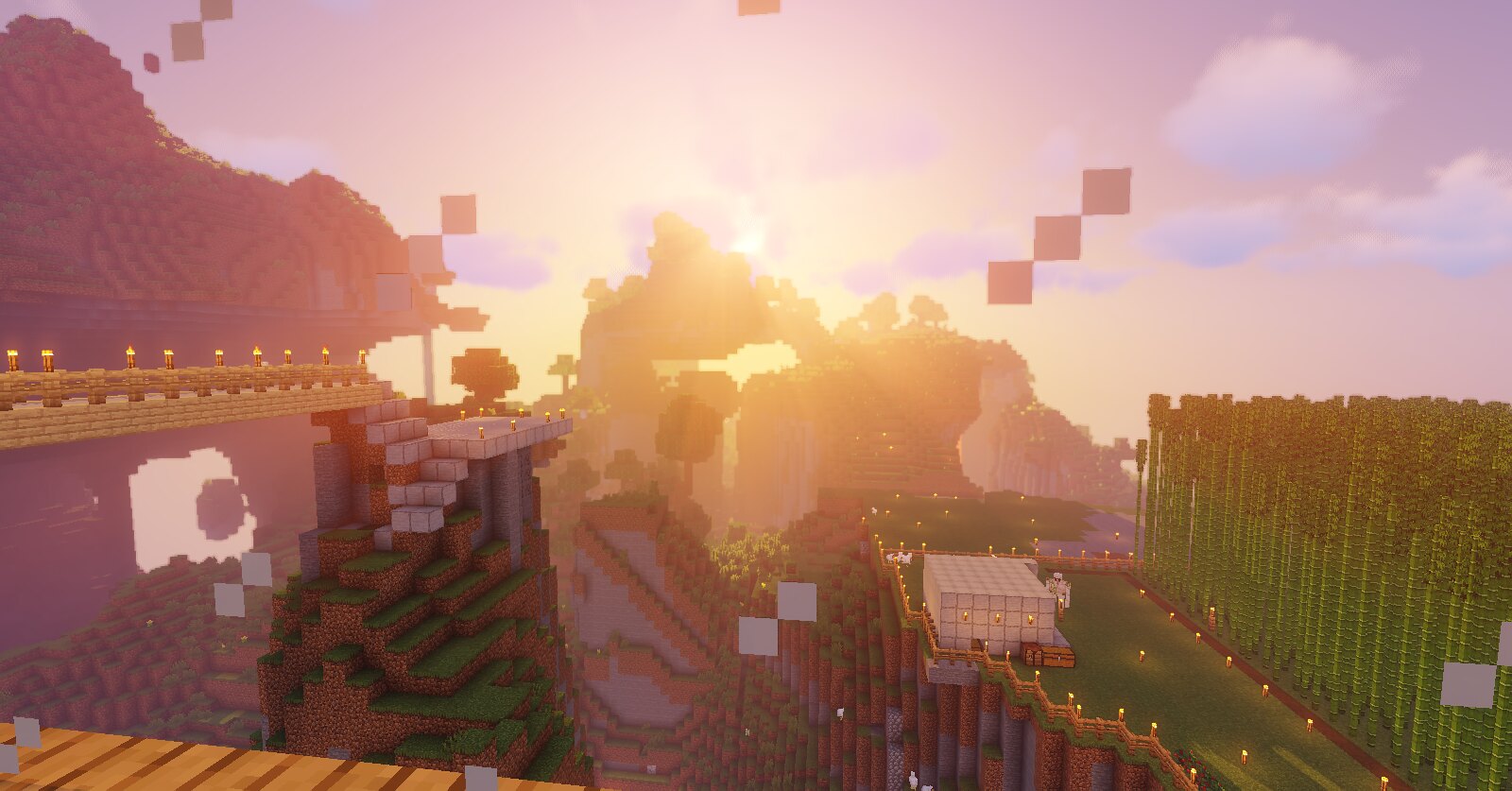This digitally created scene, reminiscent of a modded or AI-enhanced Minecraft still, unfolds under a striking pinkish-orange and yellow sky, hinting at either dawn or dusk, with fluffy white clouds gathered on the right. Sunrays blur parts of the image, adding a soft, glowing effect. The foreground is a complex terrain with lush green land, resembling steps and blocky structures, suggestive of foliage and decorative elements. Towering, uniform green trees form a barrier-like block, and thin bamboo stalks rise to the left.

A prominent cube or silver square building, likely representing iron, sits among the greenery, surrounded by various structures like canyons and additional trees. Scattered lights, or torches with flickering yellow flames, illuminate pathways bordered by light tan wooden planks and fences, indicating a crafted wooden bridge extending into the landscape.

White squares, appearing like steps or windows, span diagonally across the image, enhancing the sense of depth. A walk path winds through the scene, sporadically lined with tan fence posts and burning torches. To the right, an iron golem, a mythical creature crafted from silver iron blocks, stands guard, adding a fantastical element to this vibrant and varied landscape.